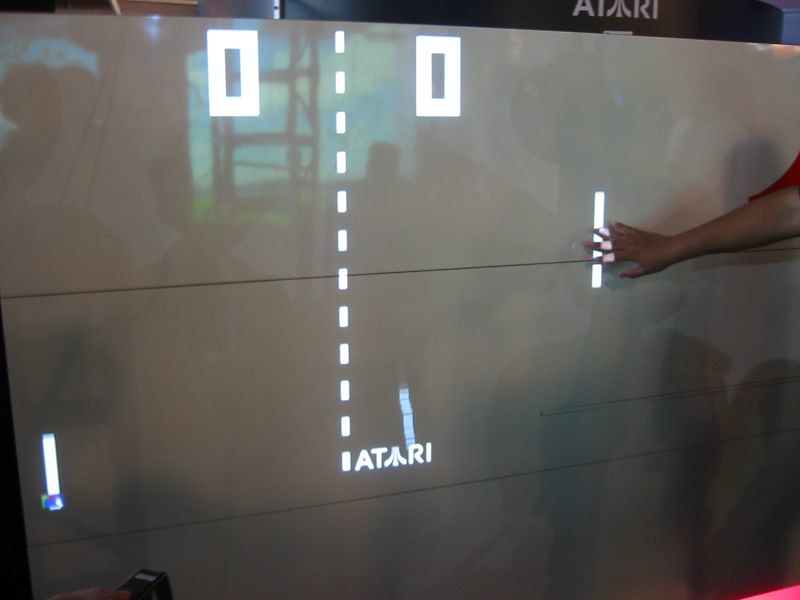The image showcases a large, reflective and shiny white projector board with projections that resemble a classic Pong game. At the center of the board, there is a vertical dotted white line running from the top to the bottom half, flanked by white zeros on both the left and right sides. The board also displays horizontal black lines. Near the bottom of the vertical line, the word "Atari" is prominently written in white, with another Atari logo visible on a black surface in the top right-hand corner. There is a hand holding a black object in the bottom right corner, and another hand, with dark brown skin and wearing a red t-shirt, is pointing to the board on the right. This person's fingers are illuminated by the projected light. The background reveals a black banner with the word "Atari" in white, and a translucent effect allows a glimpse of a blue sky with clouds and a green field behind the board.